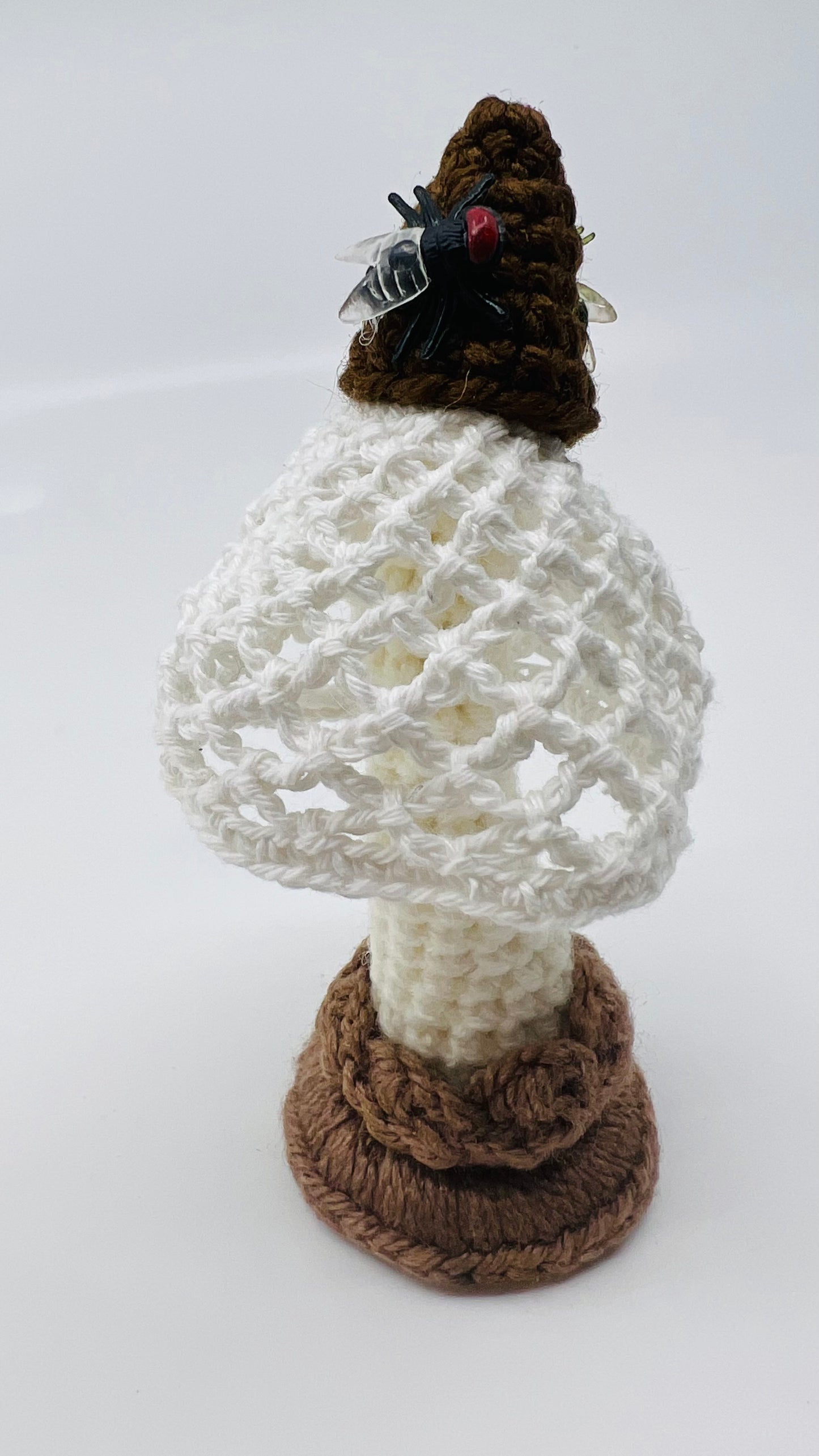This color photograph showcases a detailed close-up of a hand-knitted or crocheted piece, set against a clean white surface and background. The craft features a mushroom-like structure, skillfully created with brown and white yarn. The base of the piece is made of brown yarn, resembling a sturdy foundation, from which a white, column-like stem extends upwards. This white stem seamlessly broadens into a mushroom cap, also crafted from white yarn. Atop this cap sits a small, dark brown triangular tip, completing the mushroom appearance. The intricacy of the work is highlighted by the addition of plastic flies, one positioned at the front and another at the back of the brown tip, lending a touch of whimsy to the piece. The yarn used appears to be a winter wool material, which, despite some holes, would offer warmth. Accents of black, red, and silver from the plastic flies add to the richness of the textile art. There are no visible texts in this artistic representation, allowing the intricate crochet and knitting work to stand out entirely on its own.